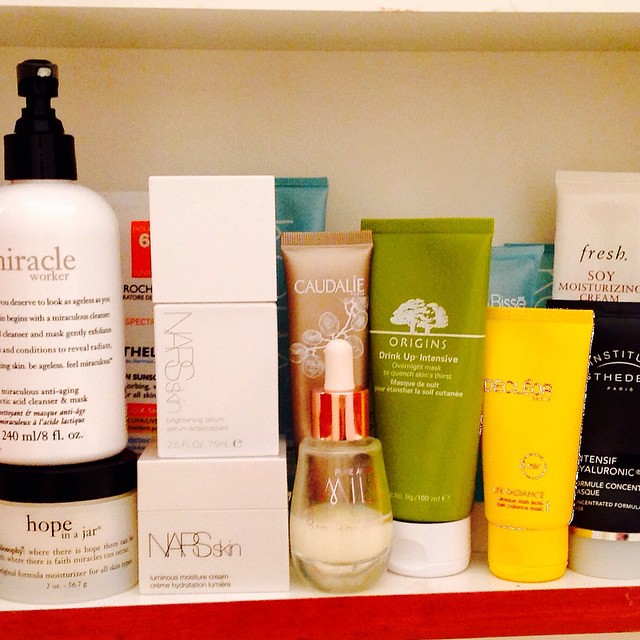This image showcases an extensive collection of beauty products meticulously arranged on a white shelf. Dominating the bottom of the frame is a red edge, adding a touch of vibrancy to the scene. On the left, there are two prominent Philosophy products: "Miracle Worker" and "Hope in a Jar." "Miracle Worker" comes in a white pump bottle with black text and a black pump, and it is positioned atop "Hope in a Jar," which features a black lid and a white jar.

To the right of the Philosophy items, a selection of NARS Skin products, still in their boxes, are neatly arranged. There is an almost clear pump, possibly an eye cream, and a bronze tube with white text labeled "Caudalie."

Next, the "Origins Drink Up Intensive Overnight Mask" stands out in its olive green tube, flanked by a yellow tube, another unidentified beauty product. Further, a black tube stands inverted, drawing attention with its contrast against the other colors. Complementing the collection, several teal tubes and a white tube labeled "Fresh Soy Moisturizing Cream" can be seen.

In the background, a glimpse of some sunscreen and an "ROCH" product marked with the number six in orange and white adds depth and detail to the assortment. This meticulously curated mix of beauty essentials highlights a diverse range of skincare and cosmetic items.